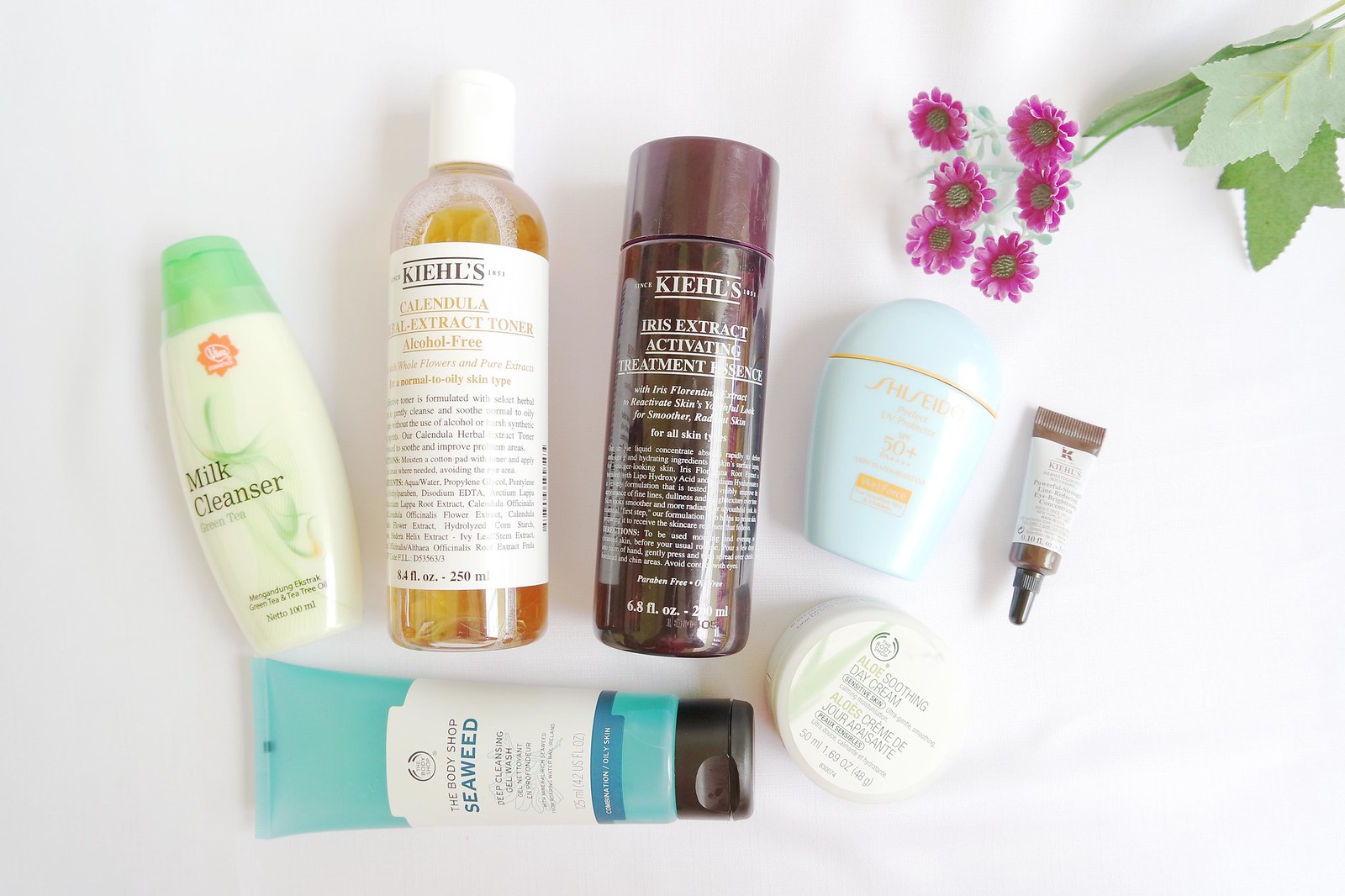The indoor photograph captures a meticulously arranged collection of skincare and health care products displayed on a pristine white surface. The arrangement consists of seven items, neatly organized from left to right.

Starting at the left, there is a milk cleanser encased in a plastic bottle. The bottle sports a cream-colored label inscribed with "Milk Cleanser" in black lettering and is topped with a green cap. 

Next to it, moving right, is a clear cylindrical bottle approximately 8 ounces in size with a white cap. The label features the brand name "KEIHL-VS" in black letters, followed by "something extract toner" beneath it.

Following this, there is another plastic bottle with a purple cap. This 6.8-ounce bottle bears the same brand name "KEHL-VS" in white lettering, with the words "iris extract" and partially obscured "activate" written below, positioned under a vertical light streak which hinders complete readability.

To the right, there is a nearly egg-shaped, pale blue item adorned with orange lettering, although the text is not legible.

Continuing, there's a very small tube, likely around half an ounce, featuring a white label and a black cap pointing downward.

At the bottom of the image, there is a horizontally positioned blue tube with a black cap pointing to the right. The label reads "seaweed," with "The Body Shop" stated above.

To the right of this, a small circular container, about one ounce in size, showcases an inscription that reads "Alloy Soothing."

In the upper right corner, a vibrant, natural element intrudes into the scene: a stem bearing six delicate purple flowers, adding a touch of organic beauty to the otherwise clinical display of products.